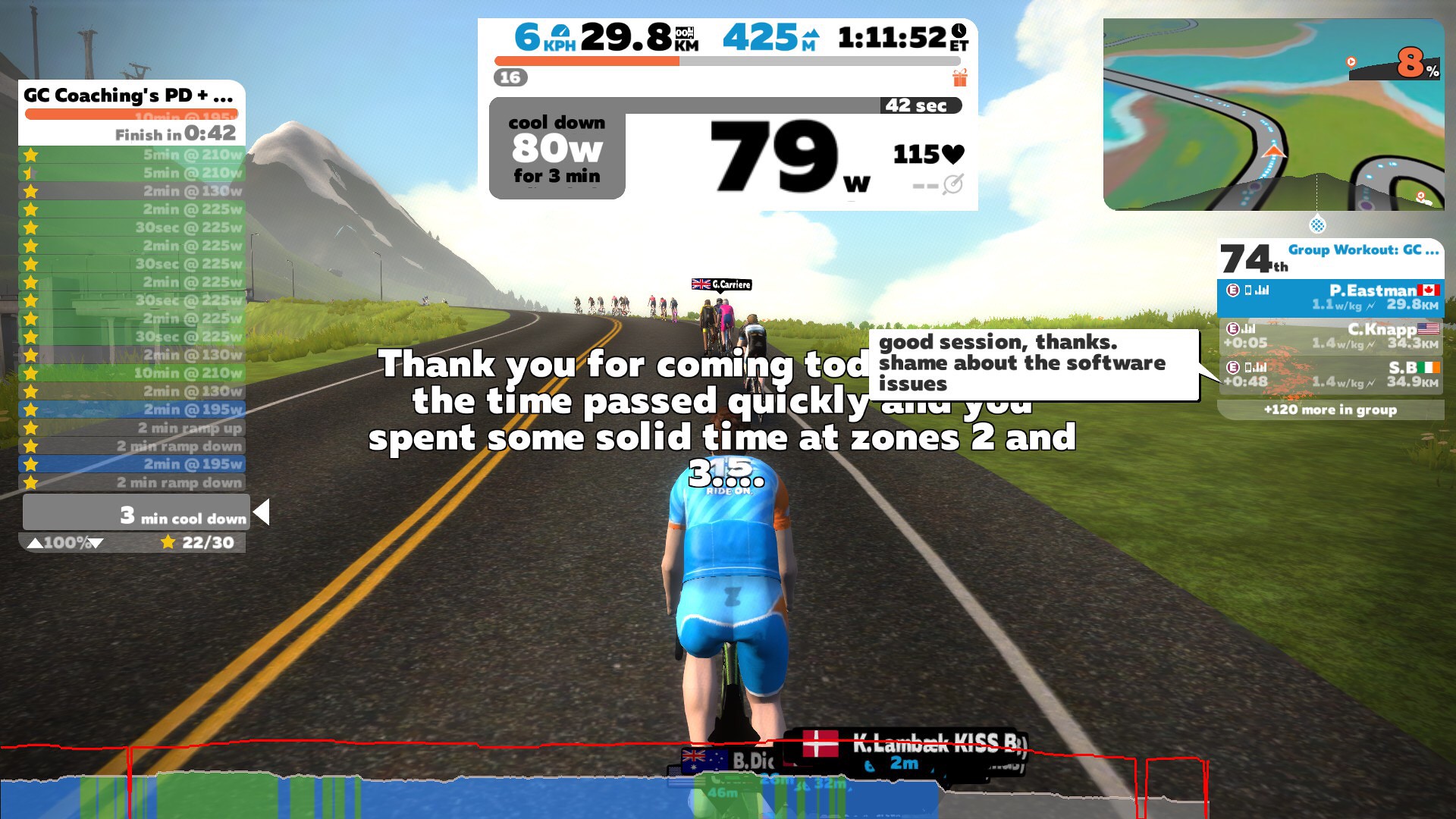The image is a detailed screenshot from a virtual cycling training game or software, possibly resembling platforms like Peloton, where players participate in a simulated cycling race. At the forefront of the race, a cyclist is prominently seen wearing a blue jersey. The screen is rich with data, beginning with a central bold text that says, "Thank you for coming today. The time passed quickly, and you spent some solid time at zones 2 and 3." This indicates the cyclist's engagement level.

On the left side, a table displays the finishing points for each player, including time taken to complete the race. The center top shows metrics like speed (6 km/h), total distance (29.8 kilometers), and time spent (1 hour, 11 minutes, and 52 seconds). Below these stats, there's mention of a cool down phase at 80 watts for three minutes, with the current heart rate at 115 beats per minute.

The top right features a dotted map, indicating the positions of various cyclists within this virtual environment. Below the map, a dialogue box reads, "Good session. Thanks. Shame about the software issues," suggesting in-game messaging or chat among users. The overall color scheme includes green, gray asphalt, and blue for the jersey, highlighting the immersive visual details. The background scenery suggests an open road with hills, enhancing the realistic experience of a cycling race.